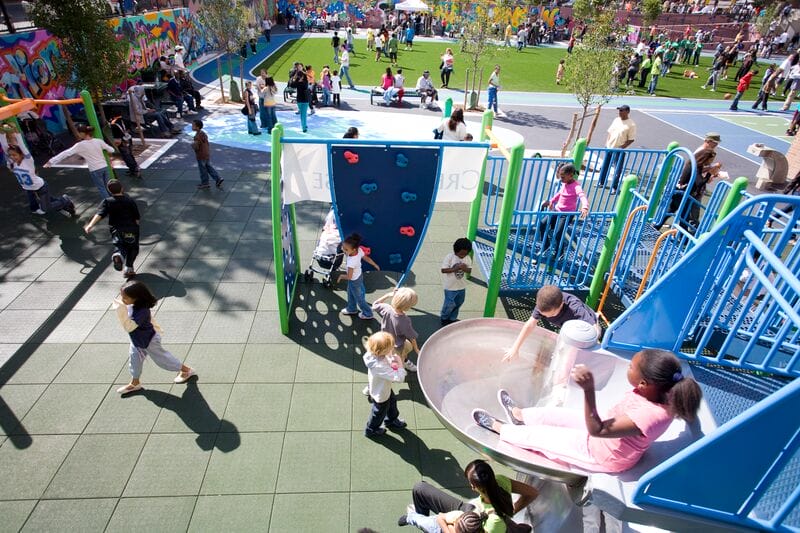The image captures a lively city park bustling with activity on a bright, sunny afternoon, likely a weekend. In the foreground, a vibrant children's play area teems with around twenty children of diverse ethnicities, engaging in various activities with visible joy. The playground features colorful equipment, including blue and green jungle gyms, a uniquely pink circular slide, and a rock wall. The ground is covered in what appears to be a green mat, designed to absorb shock, possibly made of a plastic material resembling stone tiles.

Surrounding the playground, there are stimulating murals with artistic graffiti in shades of red, blue, and green, adding a layer of visual interest and creativity. To the left, colorful walls enclose the area, enhancing the playful atmosphere.

In the background, a lush green space extends, featuring a walking or running track encircling a grassy area. Parents and guardians can be seen chatting together or keeping an eye on their children, creating a communal, family-friendly environment. Nearby, some people are engaged in a game of basketball, and tennis courts are visible in the distance, suggesting there are varied recreational options within the park. The lengthening shadows indicate that the photo was taken later in the afternoon, capturing the warmth and vivacity of this urban oasis.